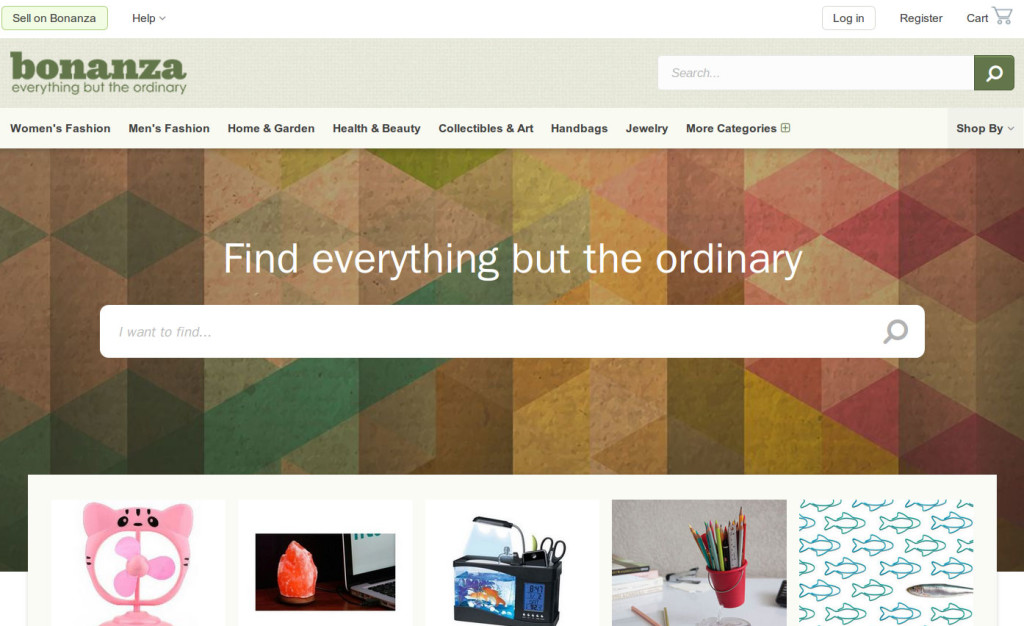The screenshot displays the interface of a website. In the upper left corner, there is a green button labeled "Sell on Bonanza". To its right, a "Help" drop-down menu is present. Moving further right to the upper corner, a "Login" button is placed, followed by a "Register" button, and a cart icon for checkout.

Directly below this top section, there is a horizontal bar stretching across the screen, characterized by a tan or gray background. On the left side of this bar, the word "Bonanza" appears in green, accompanied by the tagline "Everything but the ordinary". On the right side of the same bar, there is a search field flanked by a green search button.

Below this bar, an array of menu options spans from left to right, including categories such as "Women's Fashion", "Men's Fashion", "Home and Garden", "Health and Beauty", "Collectibles", "Art", "Handbags", "Jewelry", and an expandable "More Categories" option indicated by a plus sign. On the far right, a "Shop by" drop-down menu is available.

Further down the page, a large rectangular section filled with an assortment of colorful geometrical shapes—greens, yellows, reds, oranges, but excluding blue and purple—grabs attention. Overlaying this colorful rectangle is the phrase "Find everything but the ordinary" in white letters. Below this catchy phrase, another search bar is positioned, accompanied by a button that reads "I want to find" with a dot inside it.